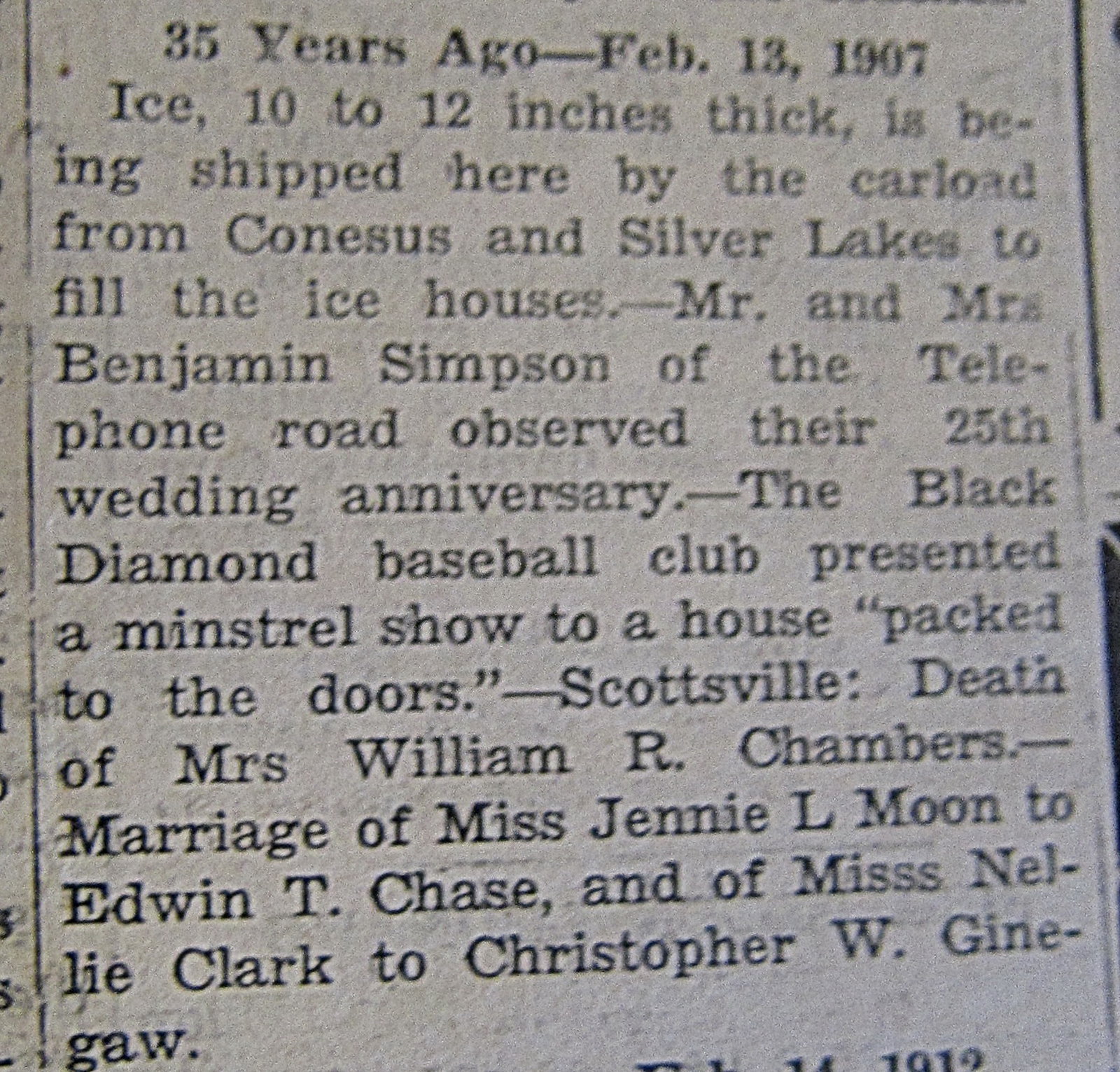The image depicts an old newspaper clipping with a white background and black text, surrounded by vertical black lines separating the columns. The headline reads, "35 years ago, February 13th, 1907." The text reports several local events: ice, 10 to 12 inches thick, is being shipped by the carload from Knessus and Silver Lakes to fill the ice houses; Mr. and Mrs. Benjamin Simpson of Telephone Road observed their 25th wedding anniversary; the Black Diamond Baseball Club presented a minstrel show to a house packed to the doors; the death of Mrs. William R. Chambers in Scottsville; and the marriages of Miss Jenny L. Moon to Edwin T. Chase and Miss Nellie Clark to Christopher W. Giengoa. The clipping captures news in a style typical of early 20th-century newspapers.